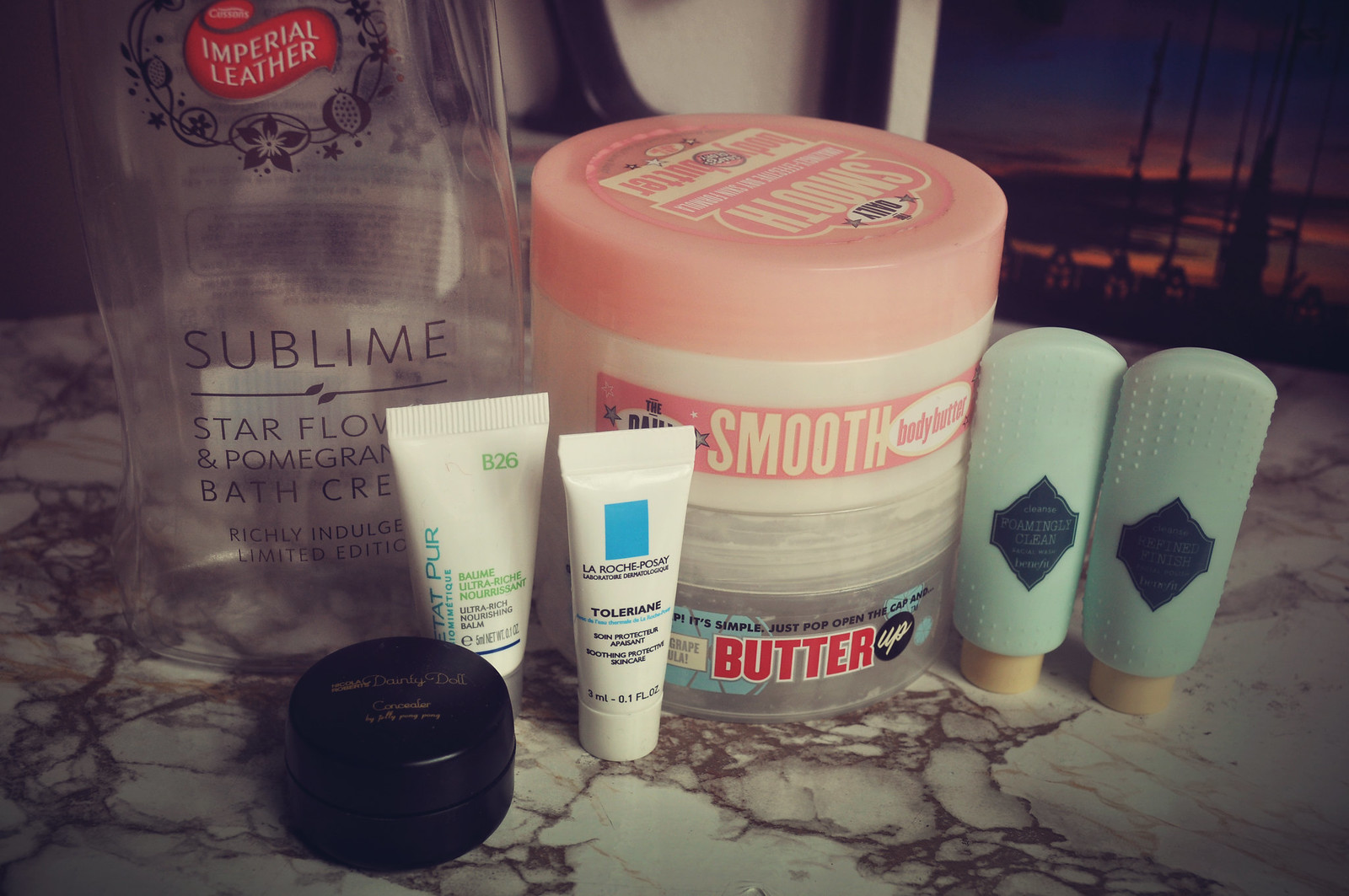This photograph depicts an array of facial and skin personal care products meticulously arranged on what appears to be a granite or marble surface. In the background, partial views of a window or door frame reveal a serene night sky with faint outlines that could possibly be railings or distant buildings. The focal point is the countertop, which is neatly adorned with a variety of product containers.

On the surface, two small, light green bottles with yellow caps, reminiscent of travel-sized hotel amenities, are prominently displayed though their labels are indistinguishable. Beside them is a large, round container with a pink lid, displaying the word "smooth" and likely containing body butter. Beneath it, another round container simply reads "butter," suggesting another type of moisturizing product.

A taller, transparent bottle is labeled "Imperial Leather Sublime Star Flake Flower and Pomegranate Bath Care Richly Indulgent Limited Edition," adding a touch of luxurious indulgence. Close by, a small white tube from La Roche-Posay, a renowned skincare brand, adds to the collection with another small white tube marked with "B26" in green. Completing the assortment is a petite black container, its contents remaining a mystery.

The staging of these items against the elegant backdrop and the tranquil night view outside creates an inviting and calming ambiance, perfect for a spa-like setting.